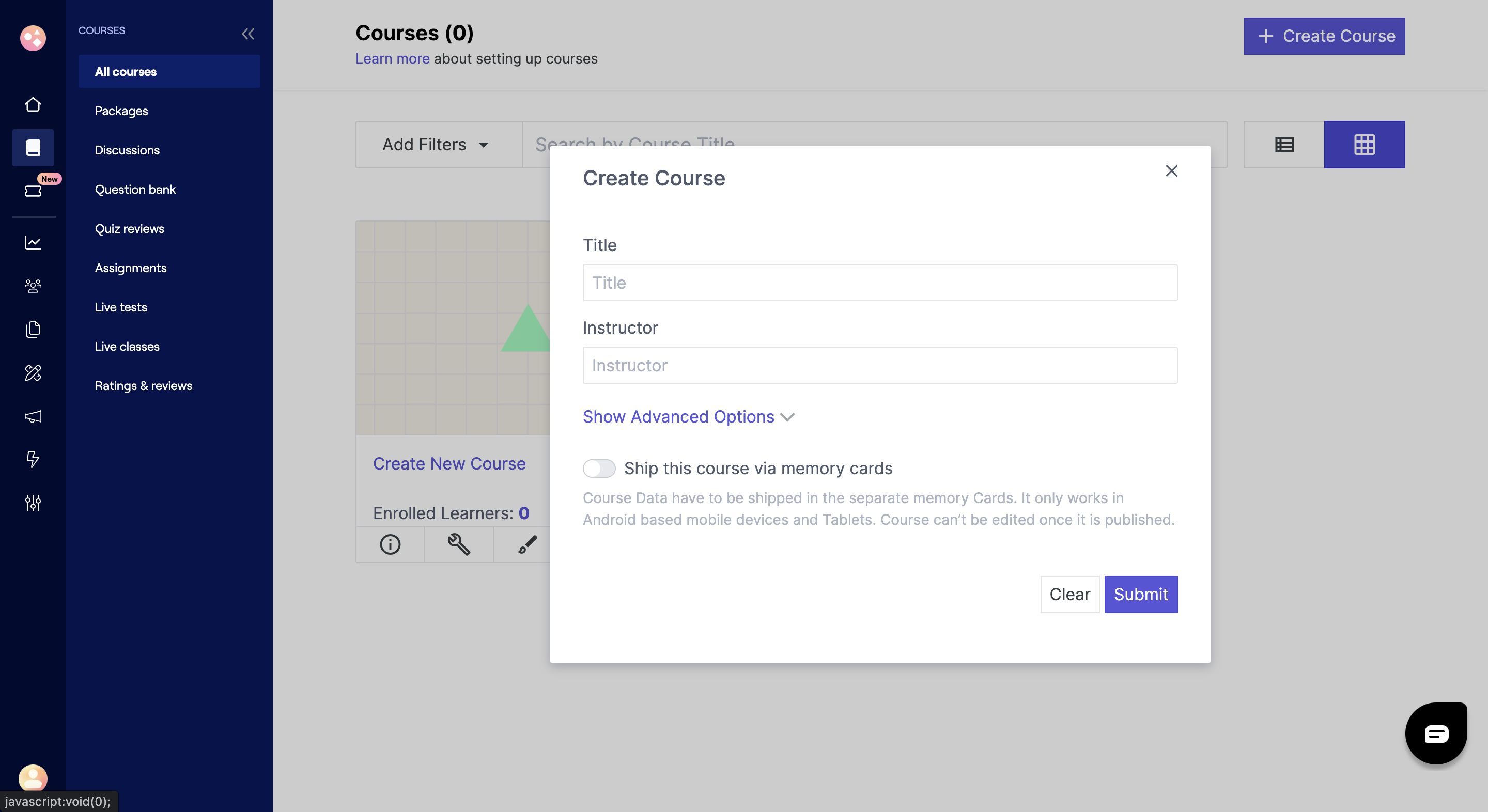The image is a screenshot of an online course creation interface resembling a college course setup. At the center of the screen is a prominent white dialog box. In the top-left corner of this box, the text "Create Course" is displayed in bold, black font. The top-right corner features a small "X" icon for closing the dialog box.

Directly below the title, there is a label that says "Title" accompanied by a white input field with a gray border, where the course title can be entered. Farther down, there is another label that says "Instructor" with a corresponding input box for entering the instructor's name.

Highlighted in blue font, the phrase "Show Advanced Options" appears below the instructor input field. Next to this phrase is a small arrow icon, indicating that it can be clicked to reveal additional settings.

Underneath the advanced options link, there is a checkbox labeled "Ship this course by memory cards," written in black font. Further clarifications in gray font note, "Course data have to be shipped in separate memory cards. It only works on Android-based mobile devices and tablets. Course can't be edited once it's published."

Finally, in the bottom right-hand corner of the dialog box, there are two buttons: one labeled "Clear" in a white box and the other labeled "Submit" in a blue box.